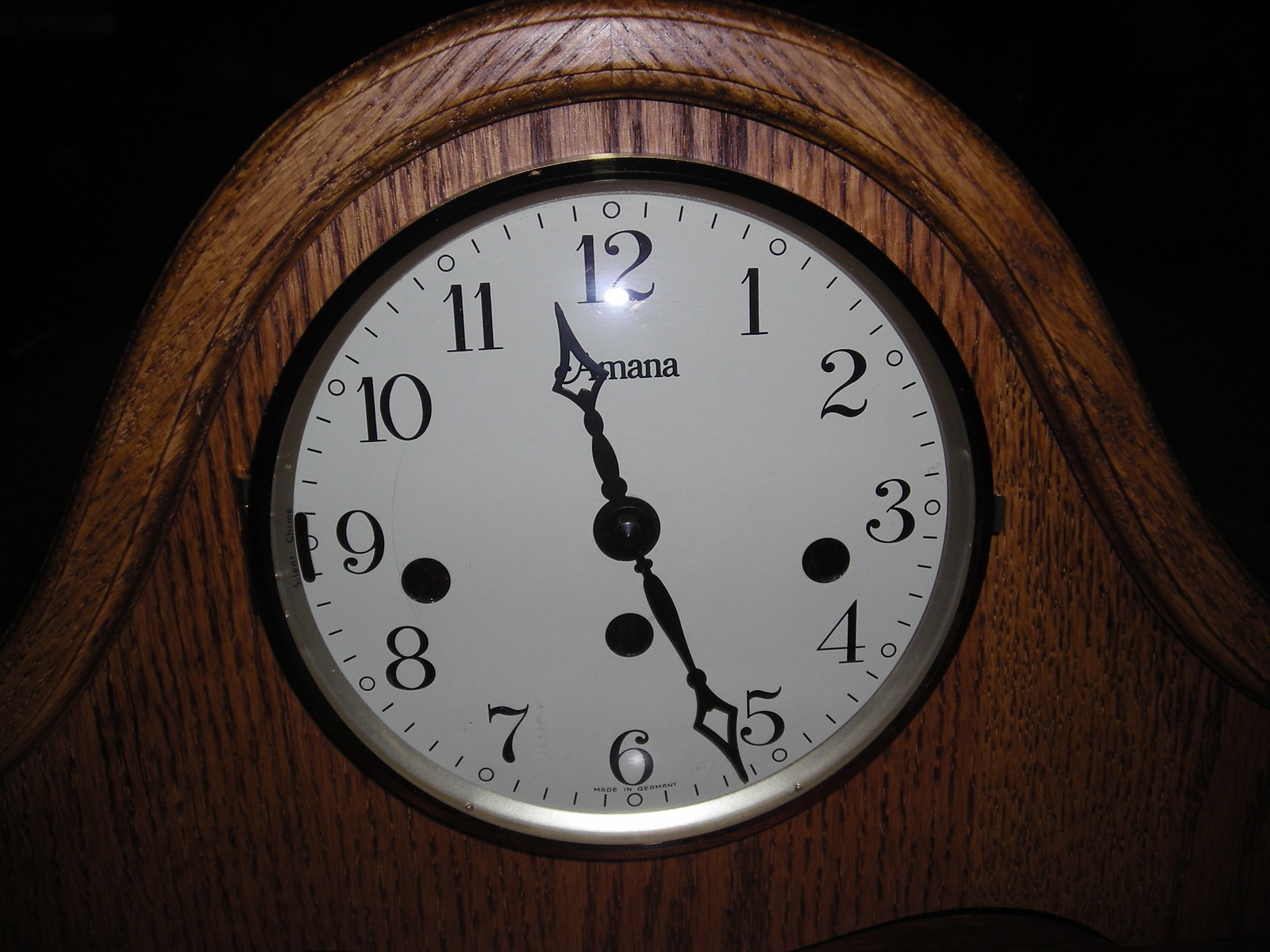This close-up image showcases a beautifully crafted clock, possibly made from oak, evident by the distinct vertical grain patterns on its main body, stained in a medium dark brown hue. The clock features an architecturally arched top, adorned with a decorative band of leather. Surrounding the clock is a trim that features grain patterns running in various directions, adding to its intricate design. 

The metal clock face is highlighted by a silver-tone ring, encircling a pristine white surface marked with black numerals from 1 to 12. Each number is accompanied by small indicators for minutes, and small circular markers positioned at each numeral. The clock displays the time 11:26, with bold hour and minute hands pointing to their respective times.

Three small black dots are visible between the 9 and 8, above the 6, and between the 3 and 4, which may serve a mechanical or decorative function. Near the 9, there is another noticeable black mark that could suggest a latch mechanism for accessing the clock face. Below the number 12, the brand name "Amanna" is elegantly inscribed, completing this refined timepiece's aesthetic.